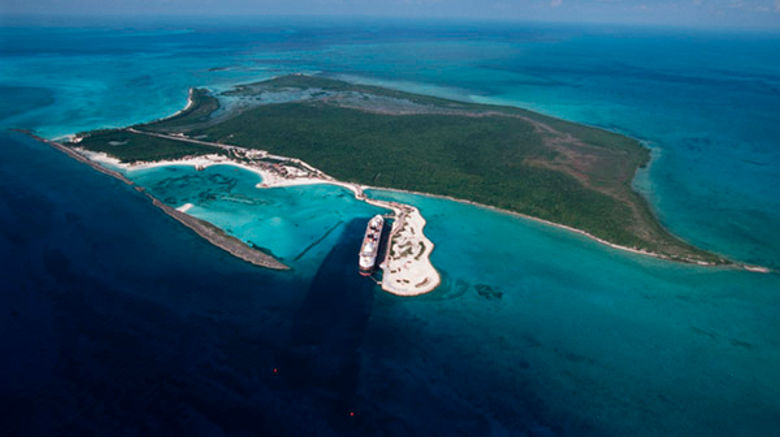This image is an aerial shot, possibly taken from an airplane or drone, capturing a rectangular-shaped island that appears largely uninhabited. The island is predominantly covered in green vegetation with some hills scattered across its landscape. The surrounding waters are a clear, deep blue. Near the coast, there is a noticeable section with white sandy beaches and some structures along the beachfront. Adjacent to the island, there is a man-made sandbar with a port where a large ship, likely a cruise liner, is docked. The ship, with several decks visible, seems to be on a stopover during a longer voyage. The scene is picturesque, with the clear day enhancing the distinct shades of blue in the sky and ocean, transitioning to darker hues towards the front of the image.